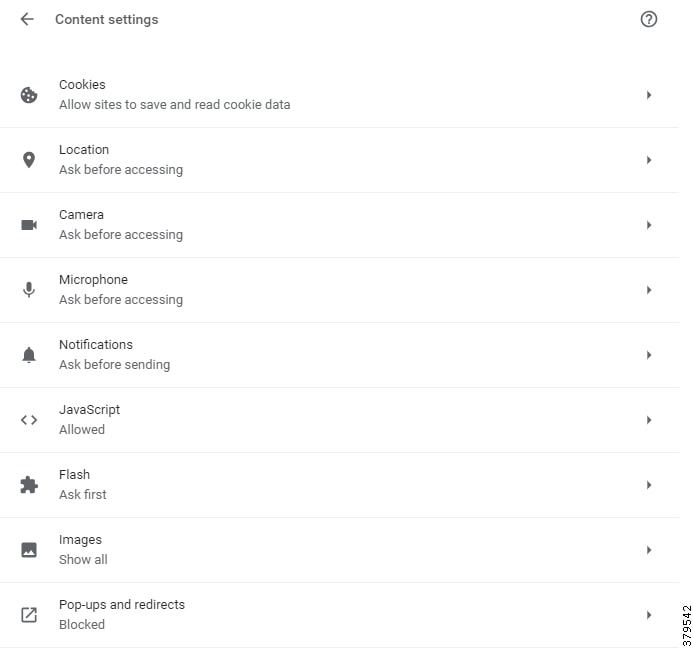The image depicts a "Content Settings" page. In the top left corner, a back arrow is displayed, followed by the bolded text "Content Settings" in a light black color. On the top right corner, there's a circle outlined in black with a white interior and a question mark centered inside it.

The body of the page consists of a neatly organized list of categories, each represented by a corresponding symbol. Each row on the left side features an icon and the category name, while on the right side, a right-pointing arrow is present for navigation. The categories and their respective settings are as follows:

- **Cookies:** An icon representing cookies with the text "Ask before accessing".
- **Location:** An icon depicting a location pin with the text "Ask before accessing".
- **Camera:** A camera icon with the text "Ask before accessing".
- **Microphone:** An icon of a microphone with the text "Ask before accessing".
- **Notifications:** A bell icon with the text "Ask before accessing".
- **JavaScript:** An icon for JavaScript with the text "Allowed".
- **Flash:** A lightning bolt symbol with the text "Ask first".
- **Images:** An icon of a picture frame with the text "Show all".
- **Pop-ups and Redirects:** An icon of a pop-up window with the text "Blocked".

Each category is separated by a thin line, maintaining a clear distinction between different settings. The icons visually represent their respective features, such as a bell for notifications and a microphone for the microphone setting.